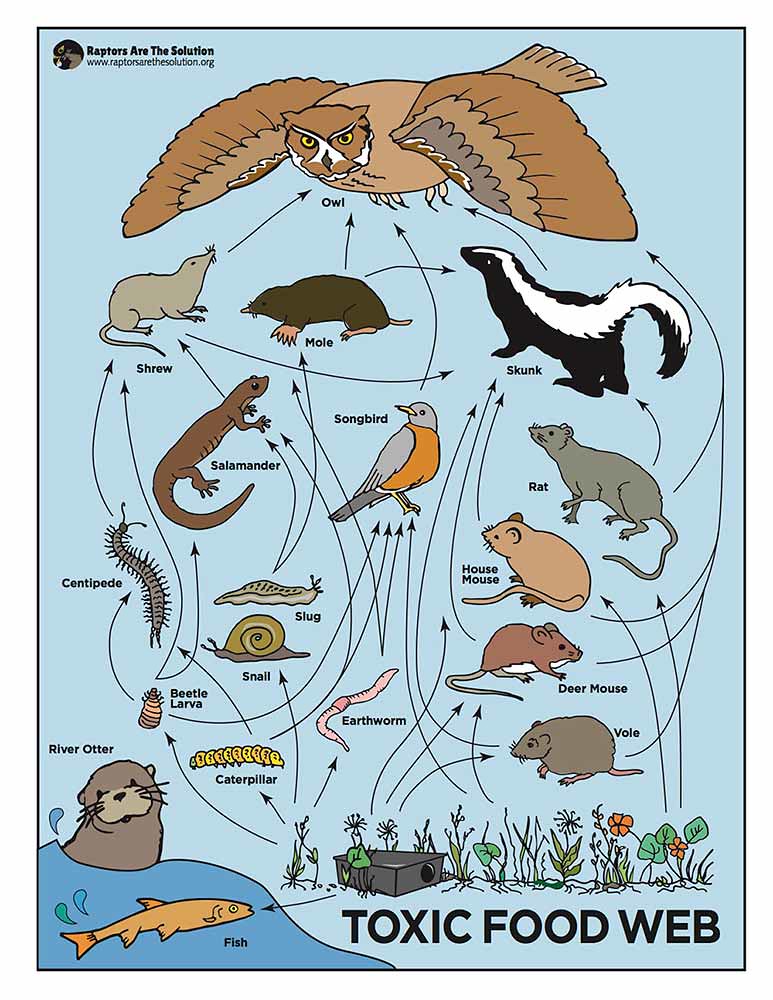This illustrated infographic, titled "Toxic Food Web" and created by Raptors Are The Solution (www.raptorsarethesolution.org), vividly portrays the complex and harmful effects of rat poison on wildlife. Featuring a cartoon-style design, the bottom right corner displays a small body of blue water with an orange fish labeled as "fish," next to a brown river otter emerging from the water. Arrows extend from a rat poison box to various organisms, demonstrating the flow of toxins through the ecosystem. 

The image details how toxic substances affect multiple species: poisoned plants and rat poison lead to contaminated caterpillars, earthworms, and beetle larvae, which are subsequently consumed by predators such as centipedes, birds, and shrews. These smaller creatures are then preyed upon by larger animals like moles, songbirds, skunks, and owls. A notable pathway shows how a poisoned vole, deer mouse, or rat might be eaten by a skunk, which is in turn consumed by an owl.

Positioned prominently at the top center is a brown owl with wide-spread wings, signifying the apex predators affected by this toxic chain, including other raptors like eagles. The poster emphasizes the widespread impact of rat poison throughout the food web, ultimately affecting top predators, and concludes with the message that "Raptors Are The Solution," advocating for awareness and a safer approach to pest control.